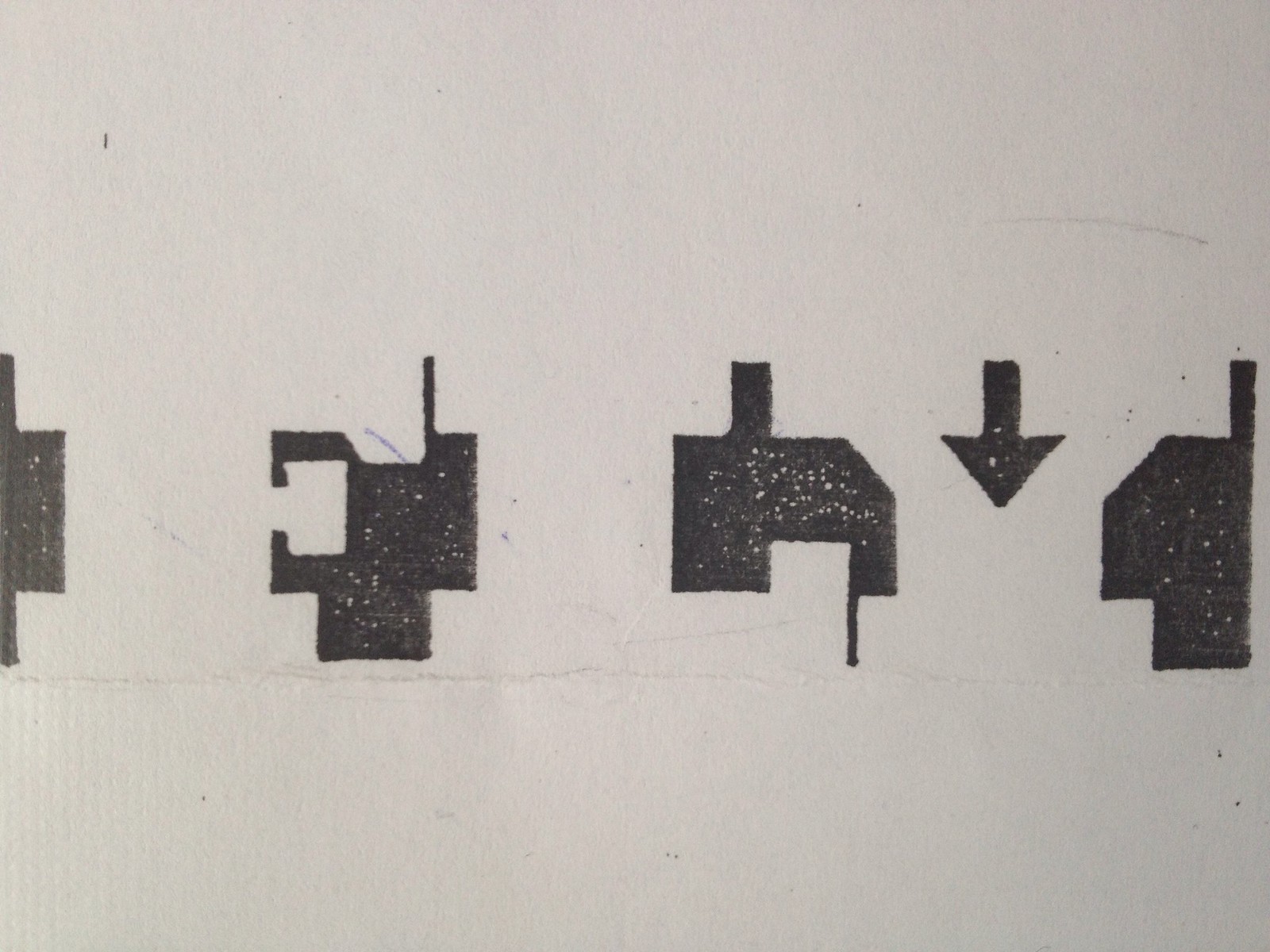The image features a series of five abstract black shapes on a white background. These shapes resemble basic outlines, somewhat reminiscent of Lego blocks, punctuated with small white specks. Upon closer inspection, the shapes take on various interpretations: one appears to resemble a sink, another a walkie-talkie, and yet another a computer component. The most recognizable among them, situated on the far right, is a downward-pointing arrow. The overall presentation has a printed, possibly aged appearance, suggesting it might be an old document or sheet related to early computer graphics or input information.